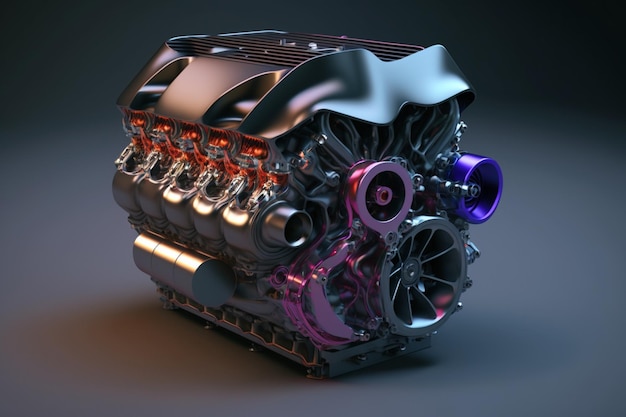The image showcases an AI-generated, intricately designed engine, seemingly a 10-cylinder V8 model, depicted at an angle against a gray background. The engine, primarily silver-toned and crafted from metal, exhibits various colored components—highlighting a blend of engineering and artistic imagination. The top features a smooth, plastic-looking valve cover with a wavy, almost alien design. Several key components of the engine stand out due to their unique colors: a pinkish-purple and anodized titanium section, a dark blue part on the right, red accents, and multicolored orange devices over the cylinders. There's a ducted fan at the front and a system of pulleys on the right side, conspicuously lacking connecting belts and appearing irregular in shape. On the left side, the exhaust assembly is attached to numerous cylinder exhaust pipes, and a reservoir cylindrical tank sits at the bottom left. The engine’s complex design, featuring potential 3D-printed elements, provides a visually detailed and surreal interpretation of automotive technology.